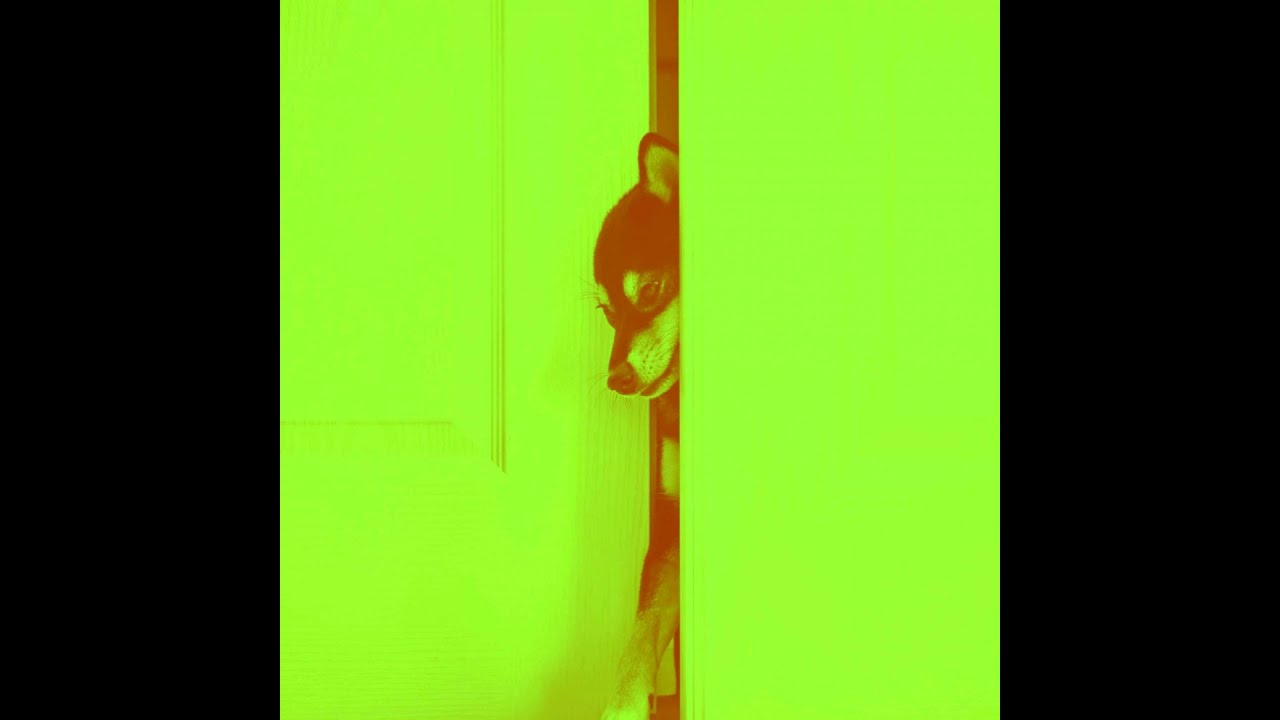In this neon green-highlighted image, we see a black and white dog, possibly a Chihuahua or a Husky puppy, attempting to squeeze through a narrow gap between an ajar white door on the left and a wall on the right. The dog's head, with its distinct black forehead and lighter-colored nose and cheeks, is visible alongside one straight ear and part of its neck. One of its paws protrudes through the gap, adding to its determined, almost contorted posture. The vibrant neon green overlay transforms the dog’s colors to shades of brown and green, evoking a surreal, artwork-like quality reminiscent of album covers. The image is framed by two black rectangles on either side, emphasizing the central focus on the dog's earnest attempt to navigate the small opening.